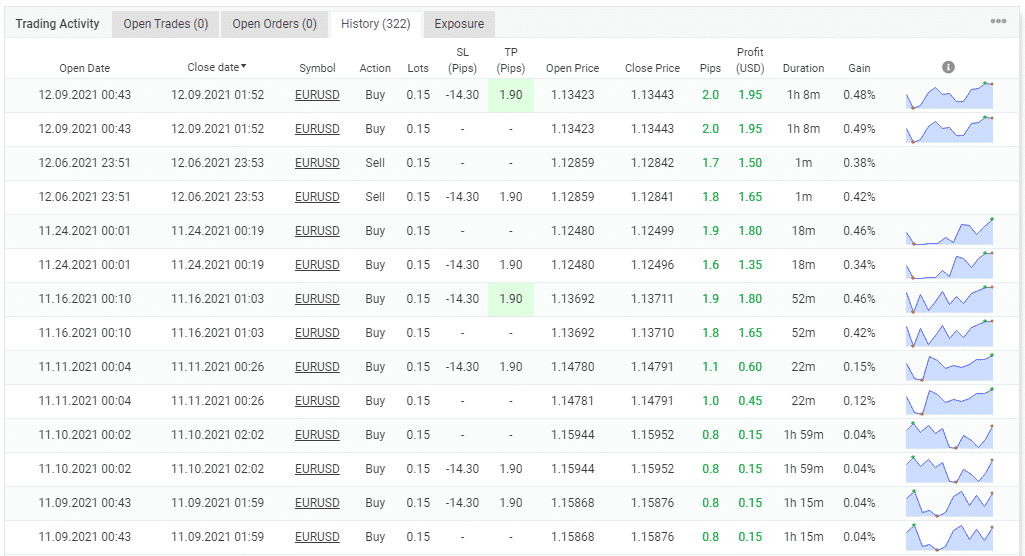This image features a detailed screenshot from a trading activity dashboard on a financial market website. The interface is set against a clean white background with thin gray lines forming rows that organize the content clearly across the page. On the right side of the screen, blue wave graphs indicate trading patterns and data. 

There are sections showcasing profit figures prominently displayed in green numbers. At the top left corner, a series of tabs provide navigational options: the highlighted 'Trading Activity' tab shows that we are currently viewing this section. Next, the 'Open Trades' and 'Open Orders' tabs both have a '0' indicating no current trades or orders. The 'History' tab highlights a significant volume with '322' items logged. Finally, there's an 'Exposure' tab.

Below these tabs, the table headers show various trading metrics including 'Open Date', 'Close Date', 'Symbol', 'Action', 'Lots', 'Pips', 'TP Pips', 'Open Price', 'Close Price', 'Profit', 'Duration', and 'Gain'. This structured layout allows for an organized and comprehensive overview of trading activities and performance metrics.